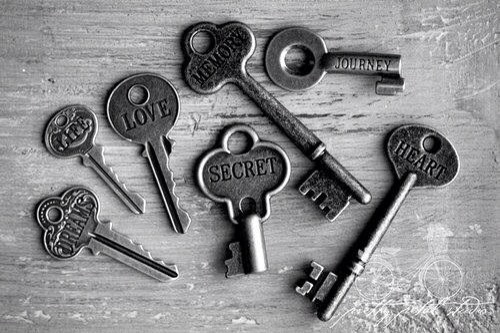This is a black-and-white photograph depicting a collection of eight intricately designed keys resting on a worn, light-colored wooden table. The keys vary in shape and style, some appearing as replicas of old-fashioned keys, complete with long rods and small pins typical of ancient designs, while others resemble more modern styles with teeth. Each key is embossed with a unique word or pattern: one says "Dreams," another "Love," a third "Secret," a fourth "Memory," a fifth "Journey," and a sixth "Heart." Additionally, there’s a key featuring a house figure at the top. The keys are arranged in a seemingly random fashion, mostly oriented with their tips pointing to the lower right. The wood of the table shows darker streaks and areas that appear very worn, adding to the timeless feel of the photograph. A signature and an unreadable logo are visible at the bottom of the image.